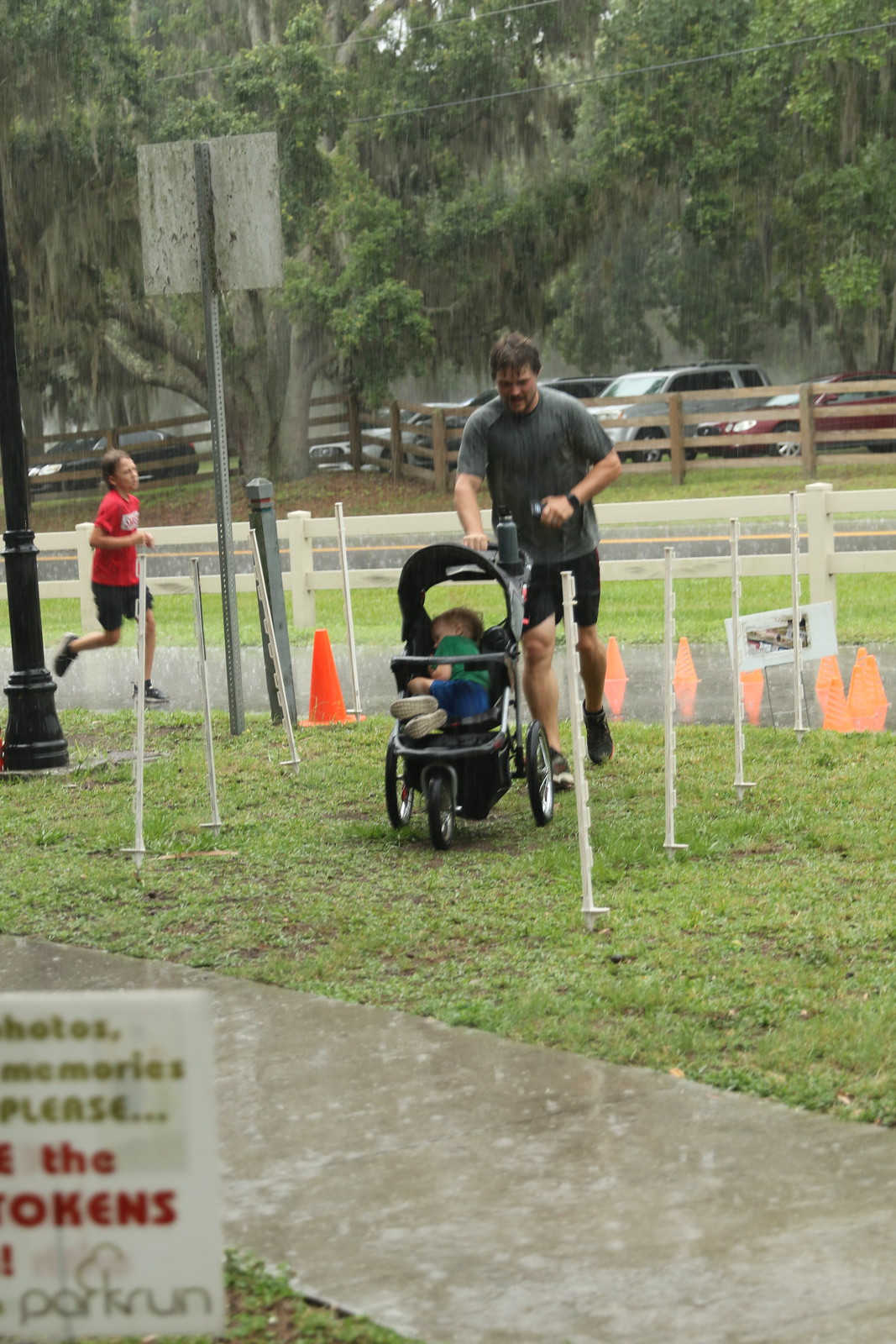In this detailed image captured on a rainy day, a man with short brown hair, wearing a gray shirt, black shorts, and a watch on his left hand, is seen running across a grassy area that leads to a wet sidewalk. He is pushing a tri-wheel stroller with a young boy inside who is clad in a green shirt and blue shorts, appearing to be asleep. Just to the left, another young boy in a red t-shirt, blue-black tennis shoes, and black shorts is running along a parallel sidewalk. A partially visible sign in the lower left-hand corner reads "park run," hinting at a possible organized race event like a 5k or 10k marathon. In the background, a wooden fence stands in front of a street lined with parked cars, bordered by numerous trees, adding a sense of depth and natural elements to the scene.